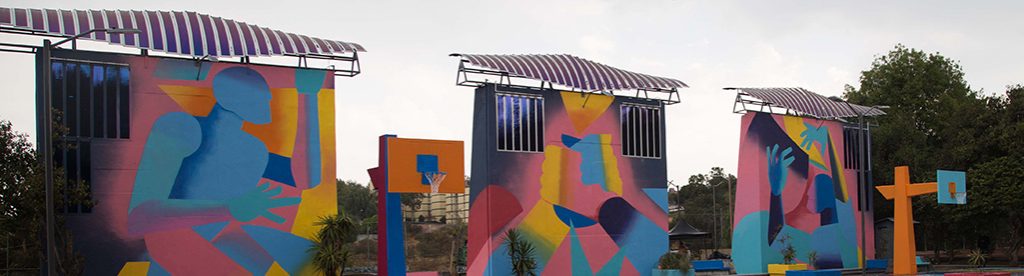This photo captures an outdoor playground scene featuring a vibrant, colorful basketball court. The court is adorned with three striking basketball-themed murals, each with an attached awning. The murals depict dynamic characters: one man poised to dribble a ball on the left, two figures engaged in a high-five in the center, and another person reaching for a ball on the right. Trees and an overcast sky frame the scene, adding a natural backdrop. The basketball hoops are uniquely designed: one with a blue base and orange backboard, and another with an orange base and blue backboard, contributing to an overall abstract and lively aesthetic.